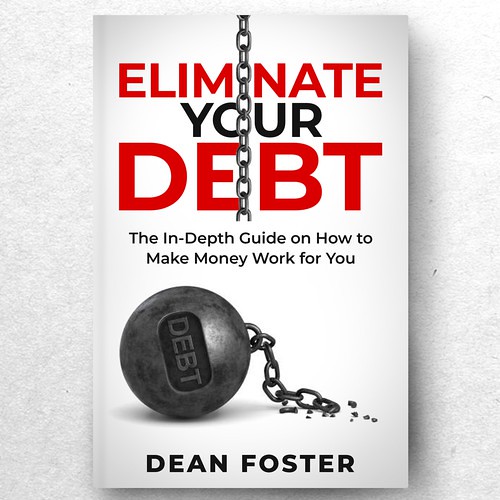This image shows the cover of a book titled "Eliminate Your Debt" by Dean Foster. The book cover features a white background with a marbled gray heathered effect. Centered slightly to the left, a large chain is prominently displayed, symbolically broken in the middle. The chain visually intersects the bold, red and black capital letters of the title, with "Eliminate" and "Debt" highlighted in red and forming the visual impression of confinement. Below the title, in smaller black text, is the subtitle, "The In-Depth Guide on How to Make Money Work for You." At the bottom, a heavy black ball with the word "Debt" written across it in dull gray lettering is depicted. The broken end of the chain is attached to this ball, reinforcing the theme of breaking free from financial constraints. The author's name, Dean Foster, is written in bold, black, all-caps lettering at the bottom of the cover. The book is positioned on a white table with a gray marbled pattern.